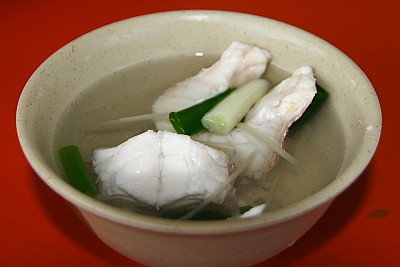The image depicts a speckled beige bowl resting on a red surface, filled with a clear broth. The broth contains chunks of white seafood, possibly crab or lobster, alongside long cuts of green scallions or spring onions and white, cylindrical root vegetables. The light in the scene suggests that the photo was taken indoors. The delicate ingredients float serenely in the clear liquid, giving the impression of a carefully prepared Asian-style seafood soup.